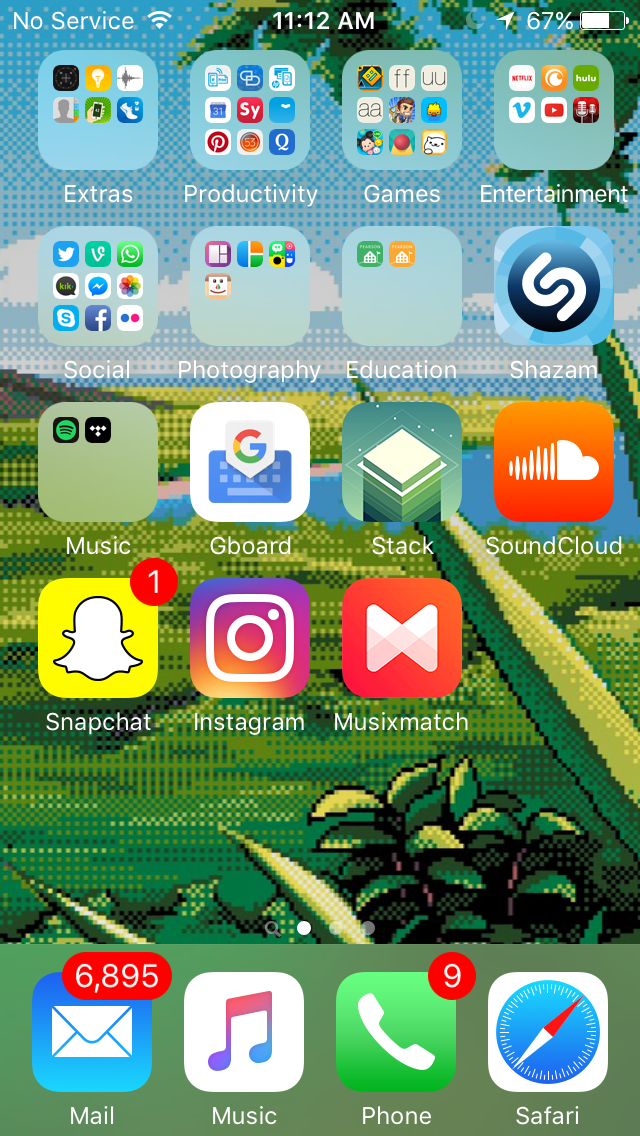The screenshot depicts the home screen of a cellphone, featuring a vibrant digital background reminiscent of an old video game. The background image is a picturesque scene of a lush jungle overlooking the ocean. At the top left of the screen, the status bar indicates "No Service." The current time, displayed in the center, is 11:12 a.m. On the top right, the battery level is shown to be at 67%.

The home screen is organized into several folders, each containing numerous apps. The folders are labeled as follows: "Extras," "Productivity," "Game," "Entertainment," "Social," "Photography," "Education," "Music," and a folder containing the Shazam app titled "Shazam." Individual apps outside of these folders include "Keyboard," "Stack," "SoundCloud," "Snapchat" (which shows a red circle with a number 1, indicating one notification), "Instagram," and "Musixmatch."

At the bottom dock, there are four frequently used apps: "Mail" (with an overwhelming 6,895 unread emails), "Music," "Phone" (showing 9 missed notifications), and "Safari."